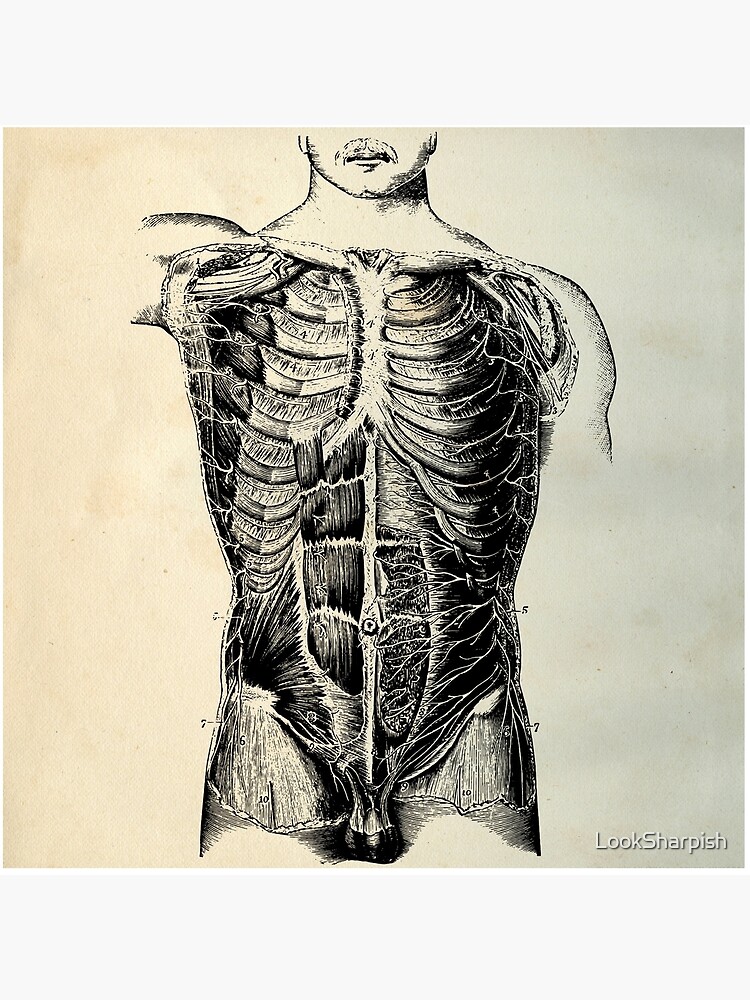This is a detailed black-and-white anatomical illustration of a man, set against an aged, weathered beige background. The drawing, which appears to have been shaded with pencil, features a human torso depicted from just below the nose down to the pelvis. The head is cropped off, showing only a mustache above the upper lip. Notably, the arms are not drawn, leaving only the shoulders outlined. The focused illustration reveals the ribcage, abdominal muscles, and the upper thighs, intricately showing the individual muscle fibers, cartilage, and veins, particularly noticeable on the right side. The depiction also includes the gonads at the bottom center. A gray border frames the top and bottom of the image, and a white watermark with the text "look sharpish" is visible at the bottom right corner, adding to the antiquated feel of the illustration.